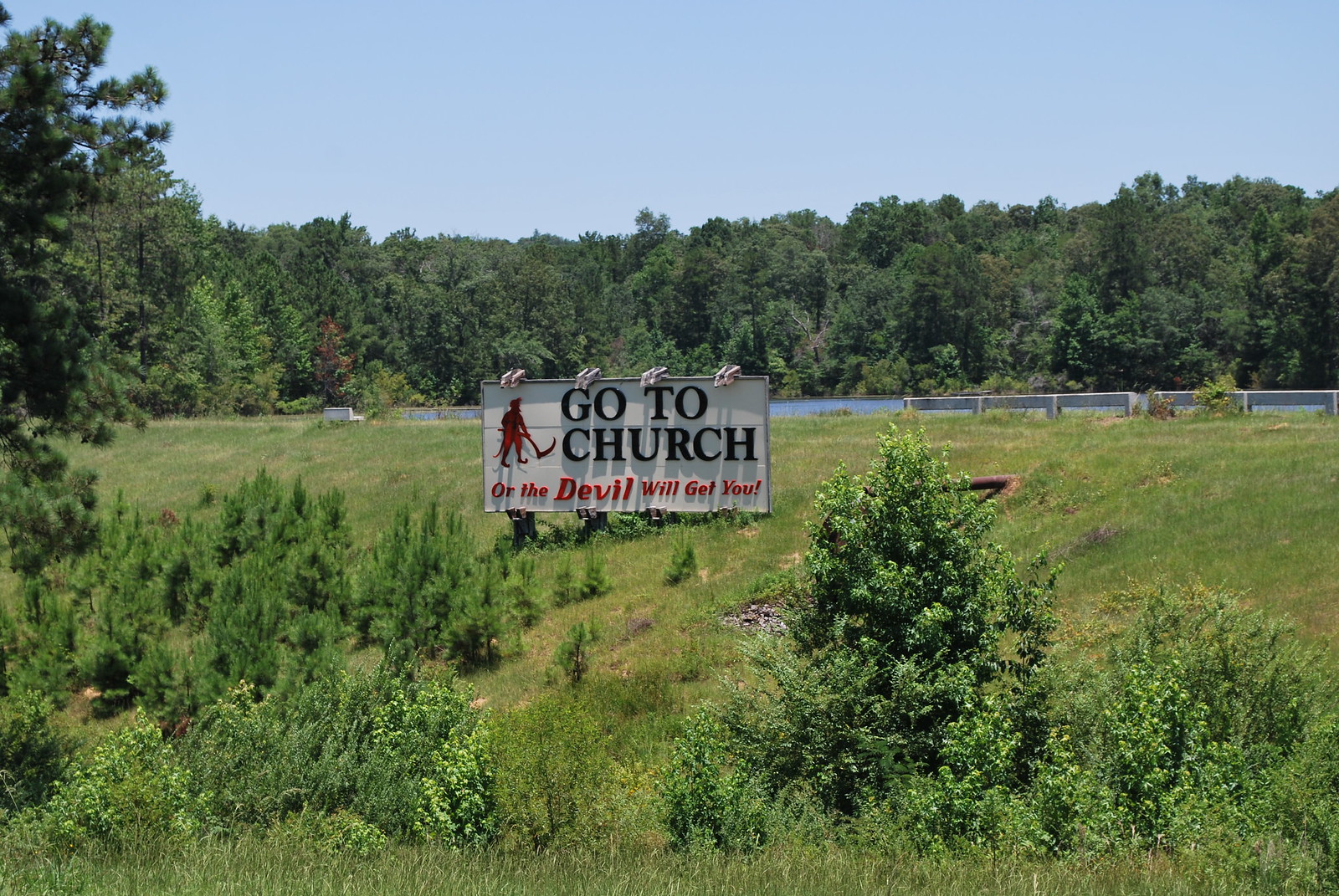The image depicts a vivid outdoor scene set against a backdrop of lush, dense forest. A light blue sky transitions smoothly into a soft white near the horizon, adding a serene touch to the setting. In the background, a variety of tall trees and shrubs rise up on a hillside, adding texture and depth. Below, a body of dark blue water glistens, presumably a lake, bordered by a quaint white fence. On the grassy hillside leading down to the water, younger trees dot the landscape, alongside the fallen trunk of an old tree.

Dominating the center is a bold, wooden sign, painted white and adorned with striking messages and imagery. The sign, which appears handmade, reads "GO TO CHURCH" in large, capital black letters. Directly beneath, in ominous red lettering, it warns, "or the Devil will get you." To the left of this text, a grim reaper or red devil character brandishes a sinister scythe, intensifying the foreboding message. The billboard also has a series of lights on top, suggesting it is illuminated at night, making its message inescapable even after dark. Nearby, a series of benches invites viewers to sit and take in the surroundings, adding a touch of humor and irony to the scene. The combination of natural beauty and stark warning creates a striking and memorable image.